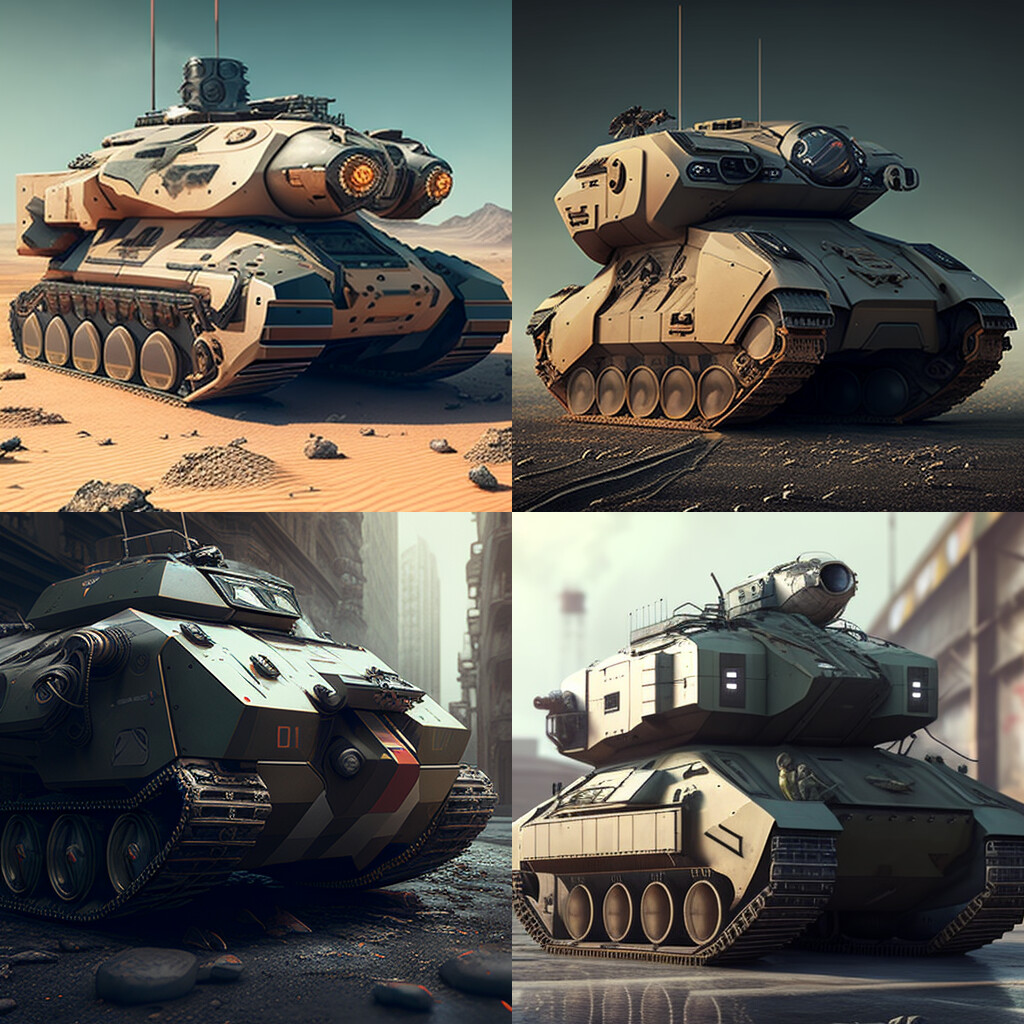This is a square image divided into four quadrants, each showcasing a digitally created, futuristic tank. The tanks manifest as sci-fi renditions possibly intended for video game design or conceptual modeling. The top left and bottom right tanks feature amber-lit elements, enhancing their advanced, dystopian appearance. The top two tanks are primarily tan, while the bottom two exhibit an army green hue, aligning them with different hypothetical environments. Each tank is equipped with tracks for movement, resembling a typical treaded base with four or five wheels encompassed by a track. Despite their similarities, each tank is set against a unique backdrop: one in a desert, another in a blackened landscape, and two in deserted cityscapes. Interestingly, there are no visible windows, but some tanks display glass-like cockpits on their smaller upper bodies. The overall color scheme is cool-toned with teal and tan tints, contributing to their offbeat, almost AI-generated appearance, characterized by a slightly unconventional shape and a sharp, futuristic aesthetic.